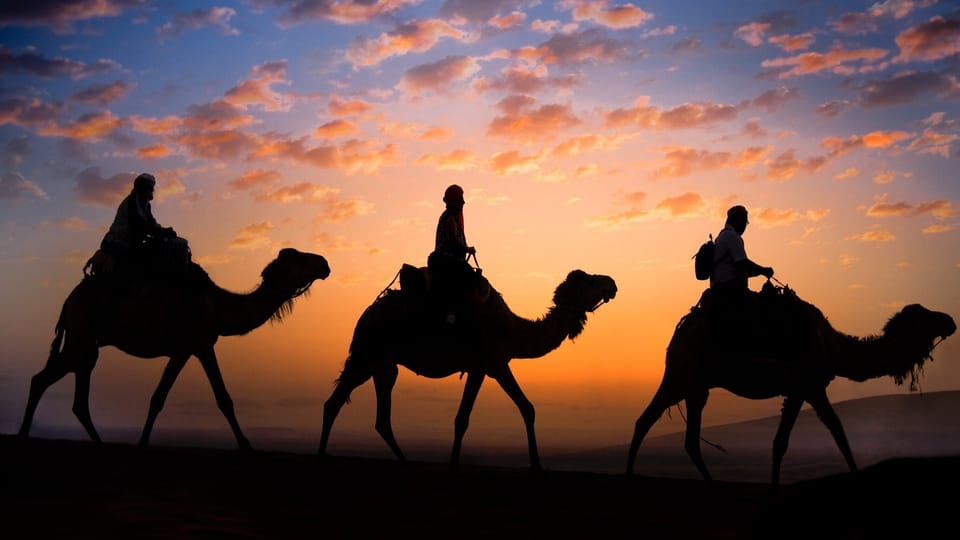In this stunning landscape photograph taken at either sunset or sunrise, three silhouetted camels, each carrying a rider, traverse a barren desert. The camels, mid-stride, are evenly spaced and follow one another towards the viewer's right. The dark foreground contrasts sharply with the vibrant backdrop, where the sky features a mesmerizing gradient from deep blue to golden orange, interspersed with cotton candy-like pink clouds. The riders, possibly men adorned in turbans, appear as black silhouettes, with the one on the far right carrying a backpack. The simplicity of the desert landscape, punctuated only by small dunes and the suggestion of a distant mountain, adds to the photo's allure, making it a perfect illustration for a travel catalog.